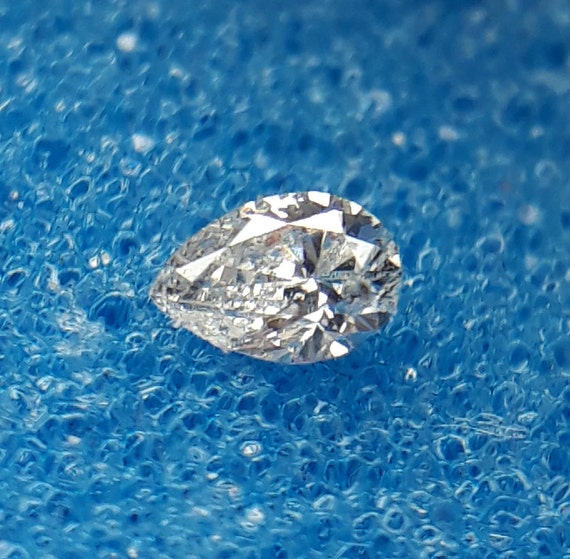This is an extremely detailed and very close-up color photograph of a large, oval-shaped diamond, lying on its side on a highly textured blue background. The diamond is exceptionally thick and shiny, with numerous facets reflecting triangles of light. The background, resembling the texture of a loofah sponge with tiny openings and round shapes, fills the entire frame and is slightly blurred at the top. The top portion of the diamond appears a bit out of focus, emphasizing its closeness to the camera.